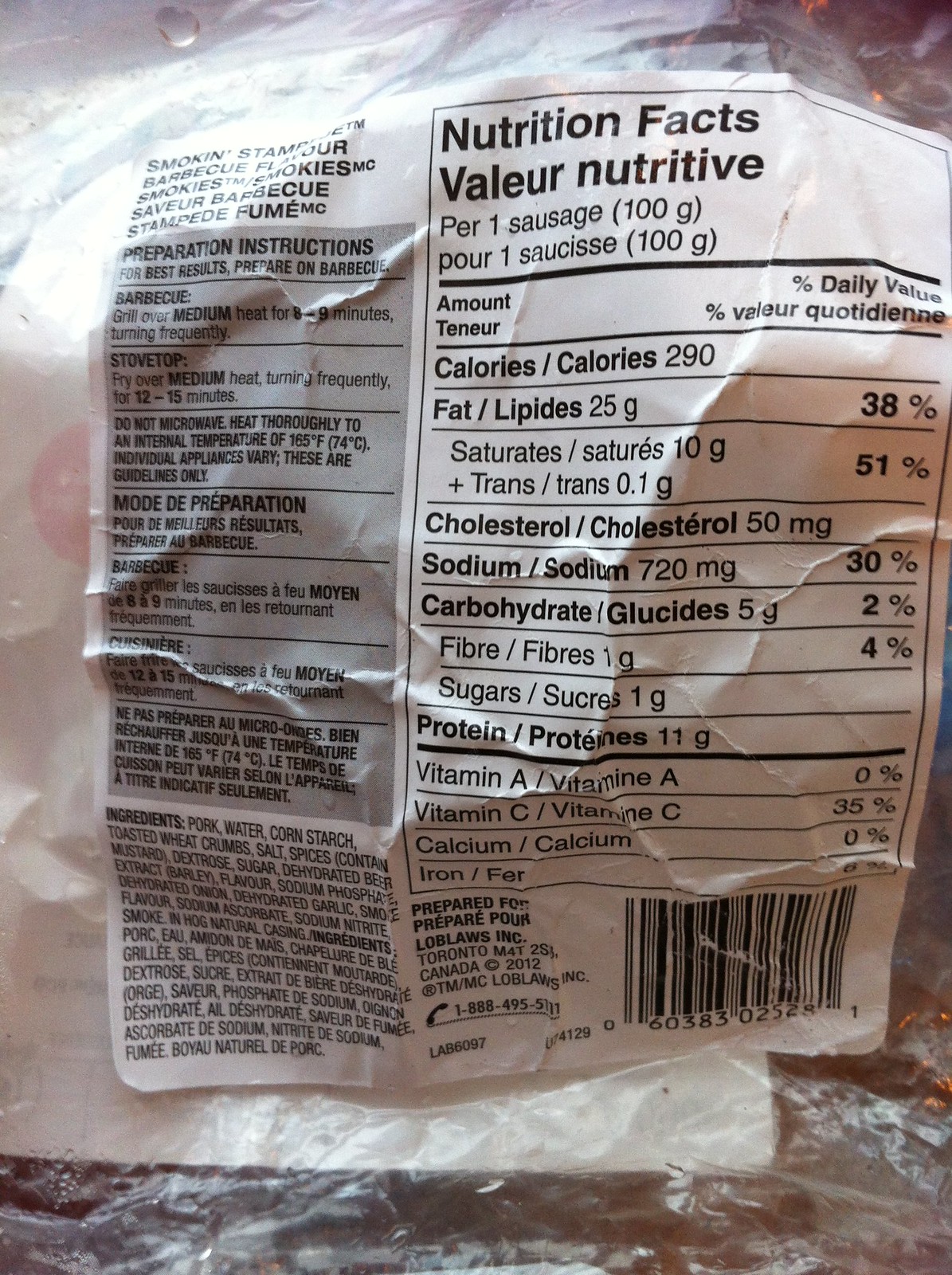The image is a photograph of a moderately lit, crinkled cellophane food wrapper with a large white label, which is partially obscured by glare from an external light source. The text on the label indicates it is a package of "Smokin' Stem for Barbecue Smokies," suggesting it contains sausages. The label is printed in both English and French, indicating it is a bilingual product. On the right side of the label, the nutrition facts for one sausage are detailed: 290 calories, 25g of fat, 50mg of cholesterol, 30% daily value of sodium, 2% daily value of carbohydrates, 4% fiber, 1g of sugars, 11g of protein, and 35% daily value of vitamin C, with no vitamin A, calcium, or iron. Below the nutritional information, a UPC code is printed in black text. The left side of the label includes preparation instructions for barbecue or stovetop cooking, explicitly stating that microwaving is not recommended, as well as an ingredients list and an address at the bottom.